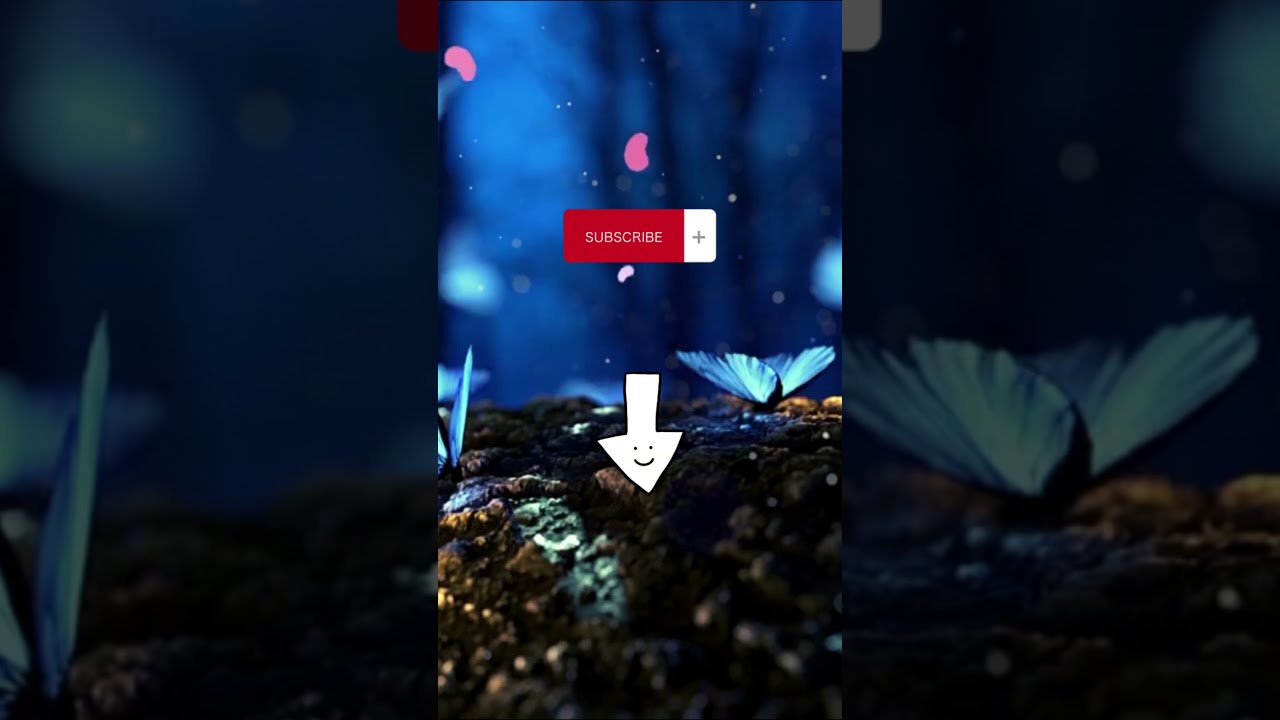This image features an extreme closeup of a rough, brown, textured ground, possibly dirt or tree bark, occupying the lower half of the center portion. The textured ground is accompanied by two butterflies with glowing, luminescent blue wings; the one on the right has its wings open, while the one on the left is partially obscured by the frame. The center photo, which only occupies the middle third of the image, is flanked by darkened, expanded versions of itself to both the left and right.

The background is a bright blue with leaf-like patterns and dark designs, further enhanced by floating pink speckles that appear overlaid, adding to the scene’s ethereal quality. Above the ground, toward the middle of the image, there's a red "subscribe" button with the word written in white, accompanied by a white box with a plus sign to its right. Below this button is a hand-drawn, white arrow pointing downward, adorned with a cartoon smiley face in black. The entire setup suggests the screenshot was taken from a mobile device, possibly from a YouTube short video, highlighting the "subscribe" call to action amidst the visually engaging scene. Multiple colors, including blue, black, white, gray, red, light green, and tan, contribute to the overall vivid composition.